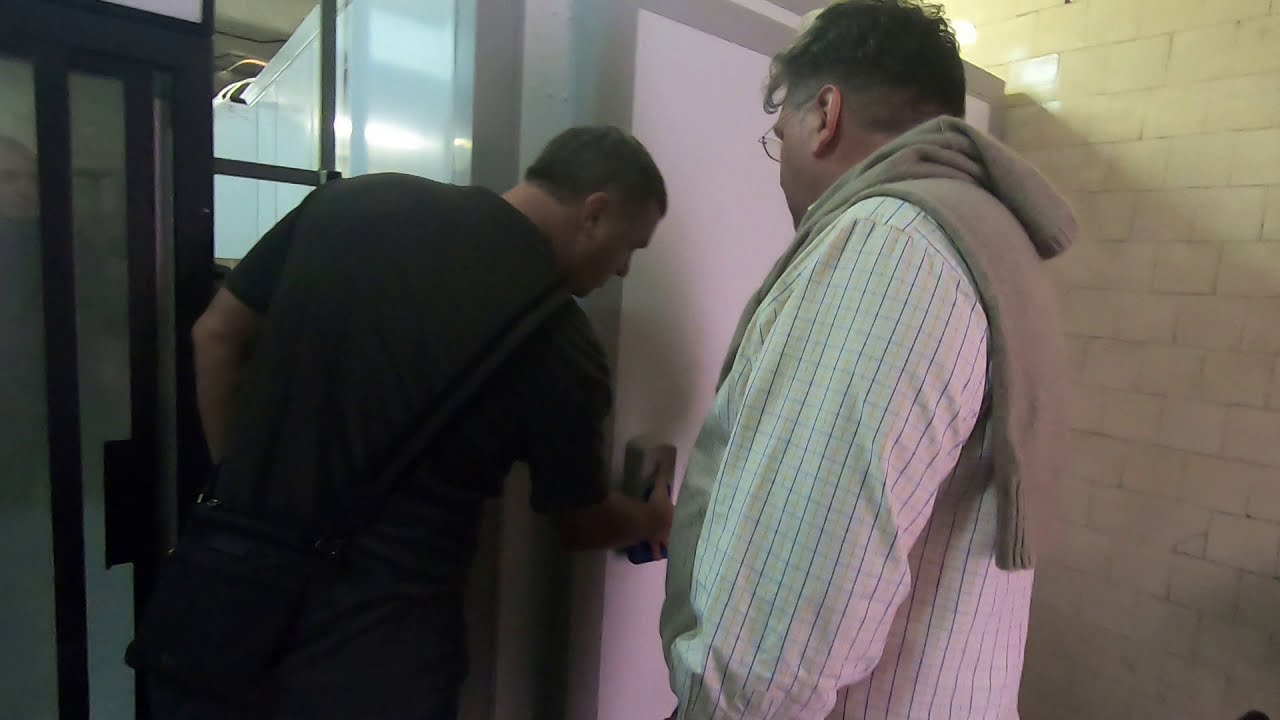In the image, two men stand with their backs facing the camera inside a building. The man on the left is bending over slightly to his right, pressing a button or touching something on a white door that has a mechanism like a keypad or lock. He is dressed in a black shirt and black pants, sporting short brown hair, and has a small knapsack slung over his shoulder. Next to him, at an angle, stands another man wearing glasses and a white and blue striped shirt with a beige sweater draped over his shoulders. They are both focused on the door, surrounded by brick walls and windows that suggest the interior of the building. The scene captures the moment as the man in black appears to be either opening the door or interacting with the mechanism, while the man in glasses observes.